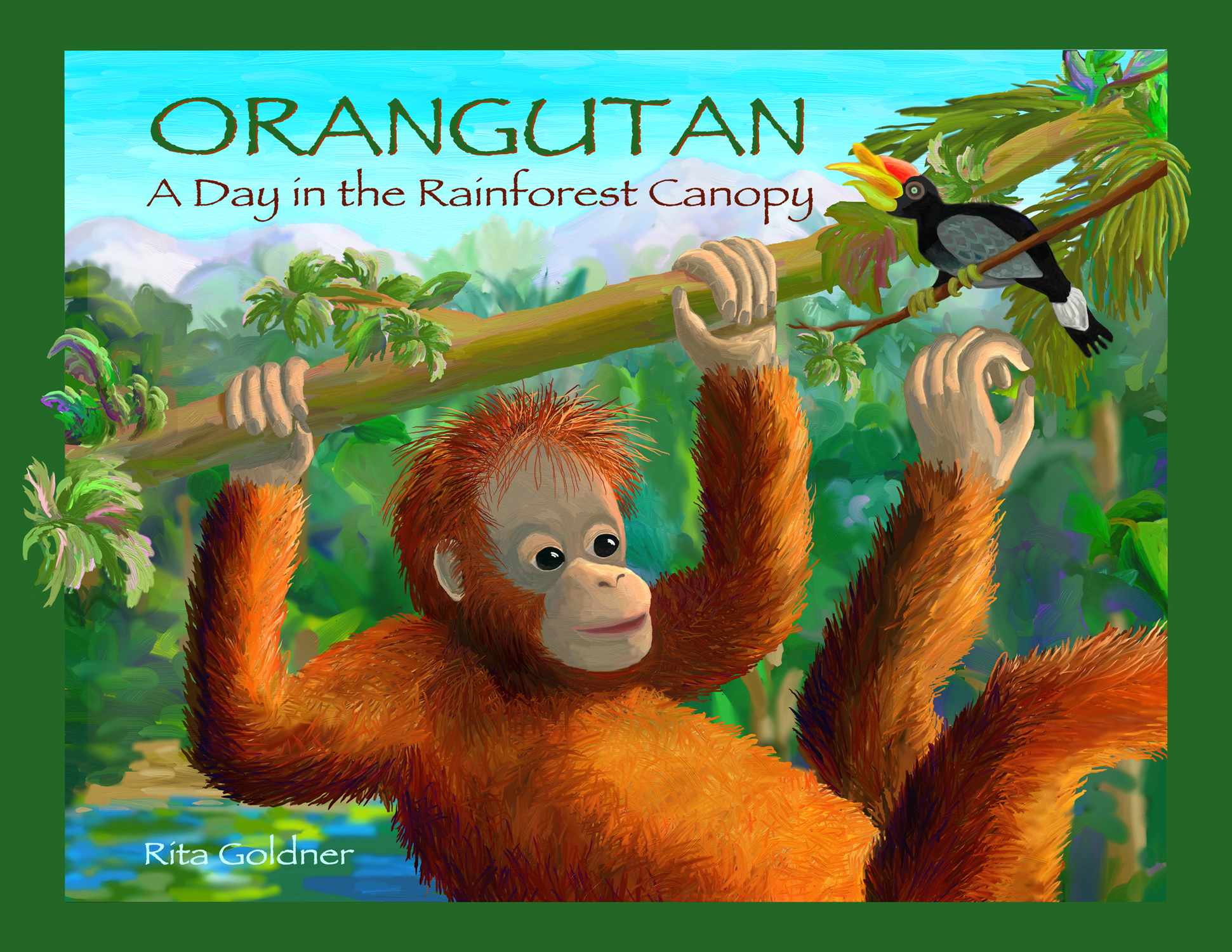The cover of the children's book titled "Orangutan: A Day in the Rainforest Canopy" by Rita Goldner is vividly illustrated, seemingly using thick, acrylic or oil-based paints. Dominated by lush, green tones, it features a young, orange-colored orangutan clinging to a greenish branch that supports scattered leaves. The orangutan, depicted from the right profile, has big black eyes, light peach-colored hands, legs, and face, and distinct red hair. A toucan with a bright yellow beak and black body perches in the upper right corner of the image. This richly detailed scene is framed by a forest green border, and a river can be glimpsed at the bottom of the cover, flowing through the rainforest canopy. The book's title is displayed in green in the upper left, alongside the author’s name, Rita Goldner, in white at the bottom left.